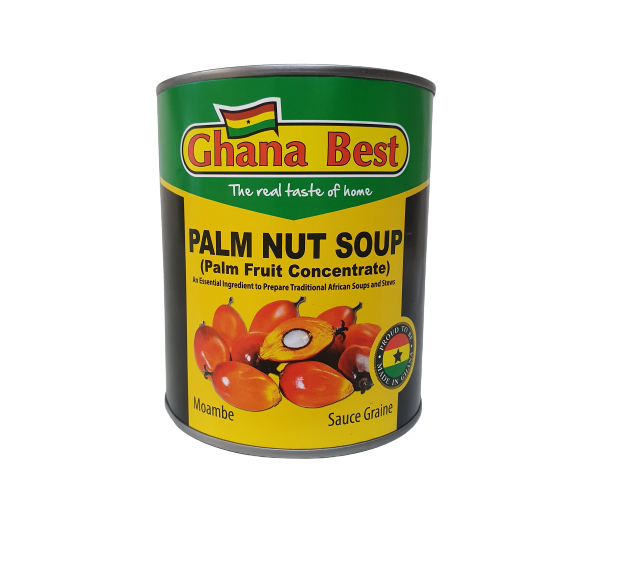This image features a can prominently labeled with the brand "Ghana Best" in bold red letters against a yellow background, which sits atop a green label at the top. Below the brand name, the tagline "The Real Taste of Home" is displayed in white letters. The central section of the label, which features a yellow background, boldly declares "PALM NUT SOUP" in all-black capital letters, followed by the descriptor "Palm Fruit Concentrate" in parentheses. Further down, the label describes the product as "Peppers Traditional African Soup", accompanied by an image of palm nuts, with one split open to reveal a white seed in the center. Adjacent to the image, the word "Moambe" is written on the left, and "Sauce Graine" on the right. Throughout the design, small circular logos feature the Ghanaian flag: red at the top, yellow in the middle with a black star, and green at the bottom, emphasizing the product's cultural authenticity. The entire label is visually framed with green at the top, black on the sides, and gray on the bottom.